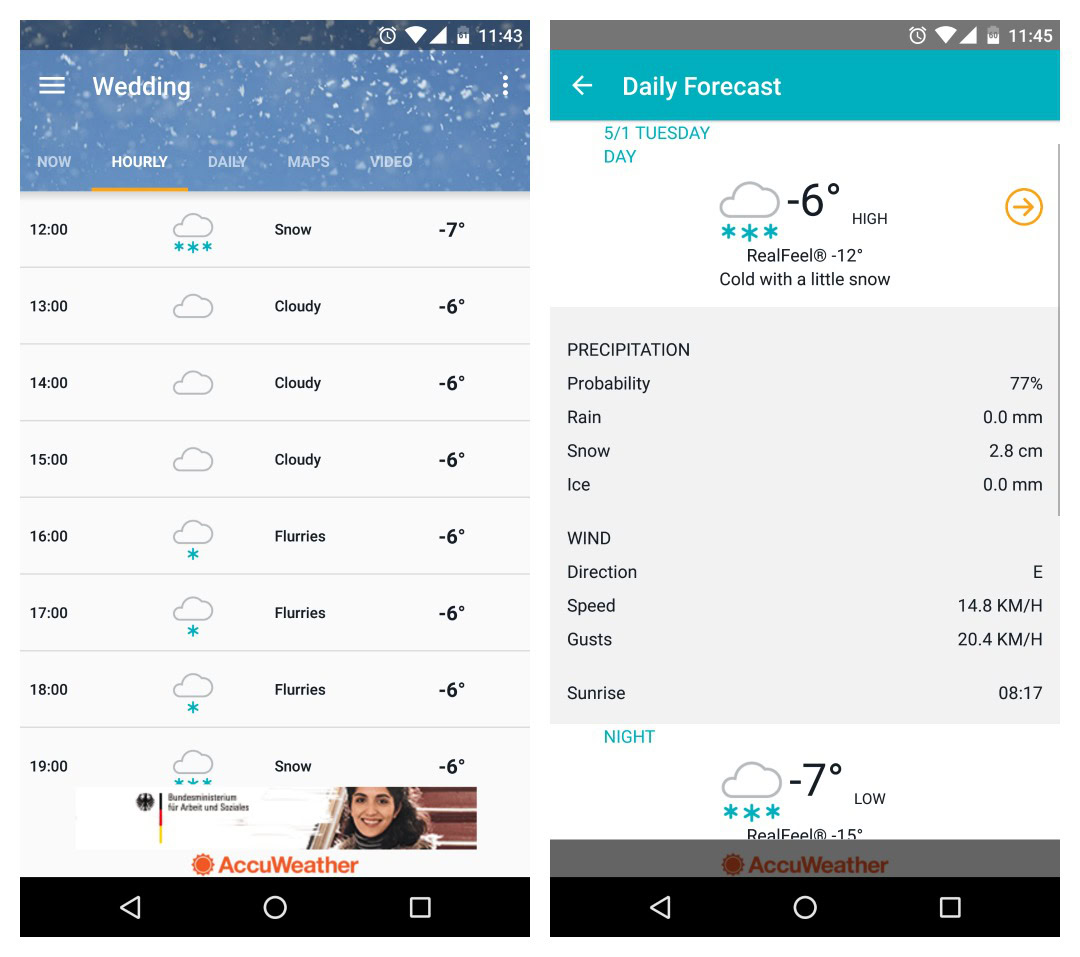This image showcases two cell phone screens displayed side-by-side, each illustrating different weather forecasts in detailed layouts.

**Left Screen:**
- **Header:** The word "Wedding" is prominently displayed at the top.
- **Forecast Layout:** 
  - Tabs: Below "Wedding" are categorized tabs: "Now," "Hourly" (highlighted), "Daily," "Maps," and "Video."
- **Hourly Forecasts (12:00 - 19:00):**
  - **12:00 PM:** Icon of a cloud with snowflakes underneath, indicating "Snow" with a temperature of -7°C.
  - **1:00 PM:** Icon of a cloud, indicating "Cloudy" with a temperature of -6°C.
  - **2:00 PM & 3:00 PM:** Similar icon of a cloud with the same "Cloudy" condition and temperature of -6°C.
  - **4:00 PM:** Icon of a cloud with a snowflake underneath, indicating "Flurries."
  - **5:00 PM & 6:00 PM:** Same condition as 4:00 PM.
  - **7:00 PM:** Icon of a cloud with three snowflakes underneath, indicating "Snow" with a temperature of -6°C.
- **Footer:** The text "AccuWeather" is displayed at the bottom of the screen.

**Right Screen:**
- **Header:** Reads "Daily Forecast 5-1 Tuesday Day."
- **Forecast Details:**
  - Icon of a cloud with three snowflakes underneath, indicating a high of -6°C.
  - Additional Information: 
    - "RealFeel" temperature is 12°C, described as "Cold with a little snow."
    - "Precipitation Probability" is 77%.
    - Rain measurement: 0.0 millimeters.
    - Snow measurement: 2.8 centimeters.
    - Ice measurement: 0.0 millimeters.
    - Wind direction: East, with speed and gust details.
  - **Sunrise Time:** Listed as 8:17 AM.
- **Footer:** The text "AccuWeather" is displayed at the bottom of the screen.